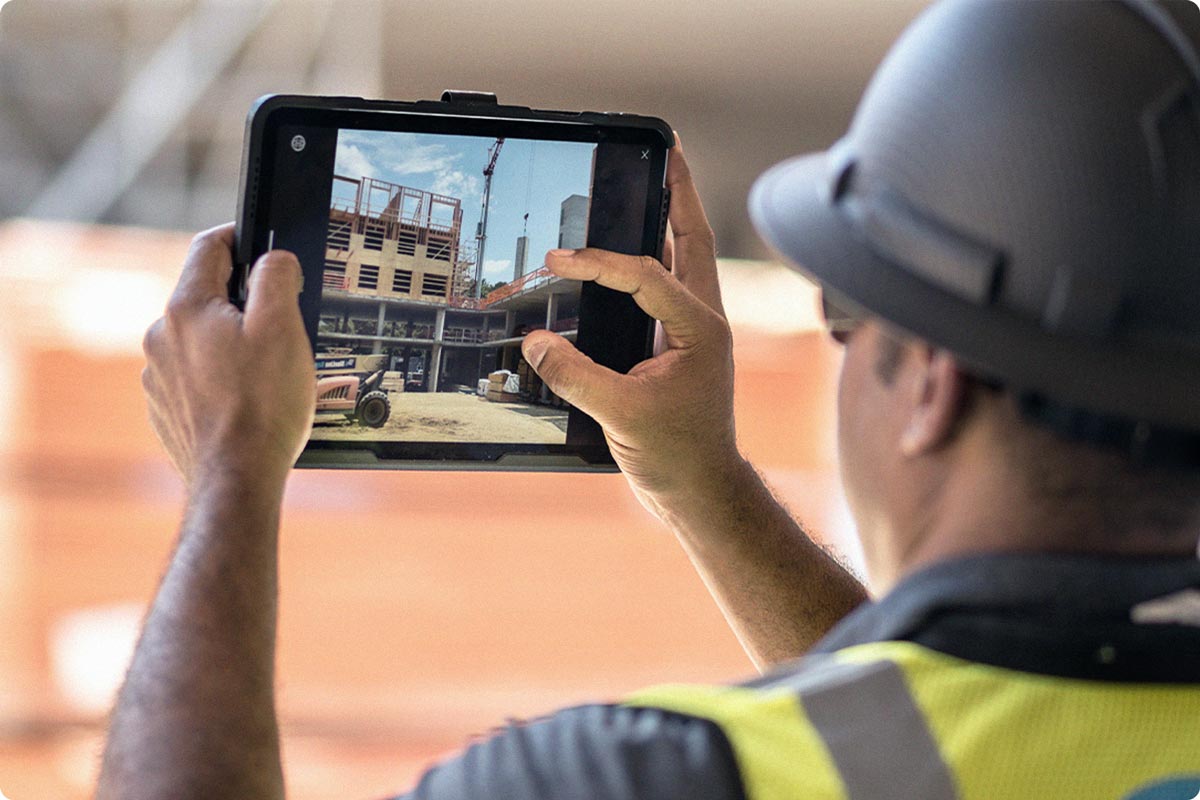In the image, a construction worker is prominently featured in the foreground. He is positioned slightly to the right, standing at what appears to be a busy construction site, which is blurred in the background, conceivably for an advertisement effect. The worker is wearing a gray short-sleeved shirt, a reflective safety vest, and a gray hard hat.

The man, possibly a foreman, is holding an iPad with both hands. His thumbs are noticeable at the edges of the device as he uses a pinching gesture to zoom in on the screen, revealing an image of the construction site with various vehicles, cranes, and partially-built concrete structures. The iPad displays a detailed view of the ongoing construction, including materials and equipment that indicate the building is still under construction.

He appears to be examining or possibly capturing the site with the iPad, which could suggest he is either viewing a live feed, potentially from a drone, or reviewing photos he has taken. The background colors show hints of orange and beige machinery and materials scattered around the construction area. The worker also has glasses, adding to his focused and professional demeanor.

The entire scene seems staged for a promotional purpose, likely highlighting the technology used in modern construction management.